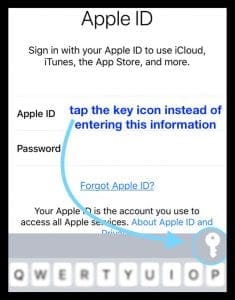Screenshot Description: The image is a screenshot of a web page with a prominent, thick black border around a white box labeled "Apple ID" at the top. Below the title, it instructs users to sign in with their Apple ID to access iCloud, iTunes, the App Store, and more. The box contains input fields for both Apple ID and password. Above the Apple ID input field, there is a blue text prompt saying, "Tap the key icon instead of entering this information" with an arrow pointing to the bottom right corner of the screen. This section is zoomed in and encircled in light blue, highlighting a silhouette of a down-pointing key. Beneath the password input field, there is a hyperlink that reads "Forgot Apple ID?" Directly below this is another line in blue text stating, "Your Apple ID is the account you use to access all Apple services" with further information about "Apple IDs and privacy." The bottom part of the screenshot shows the top row of a QWERTY keyboard, ranging from the "Q" to the "P" keys.